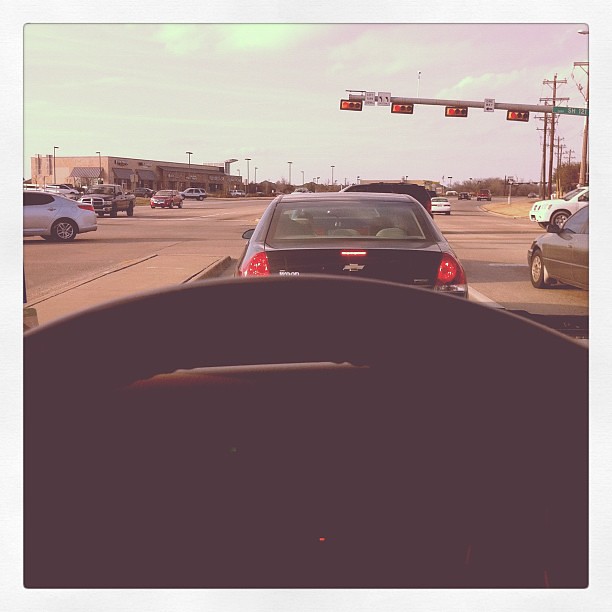In this exterior image captured with natural lighting that possesses a distinctive yellowish hue, we are given a driver's perspective from behind the steering wheel, which occupies the lower half of the frame in an all-black silhouette. Beyond the dashboard, through the windshield, extends a sprawling intersection with multiple lanes of traffic flowing in different directions. Vehicles move in both forward and perpendicular orientations, with some lanes coming in from the right side of the frame horizontally. Above, the sky appears heavily overcast, painting a gray, somber atmosphere. From the upper right corner of the frame, a sizable metal beam juts out, supporting horizontally-aligned traffic lights beneath it. The traffic signals, arranged such that the red lights sit to the far left, all display a red stop signal, suggesting a temporary pause in the bustle of the crossing traffic.